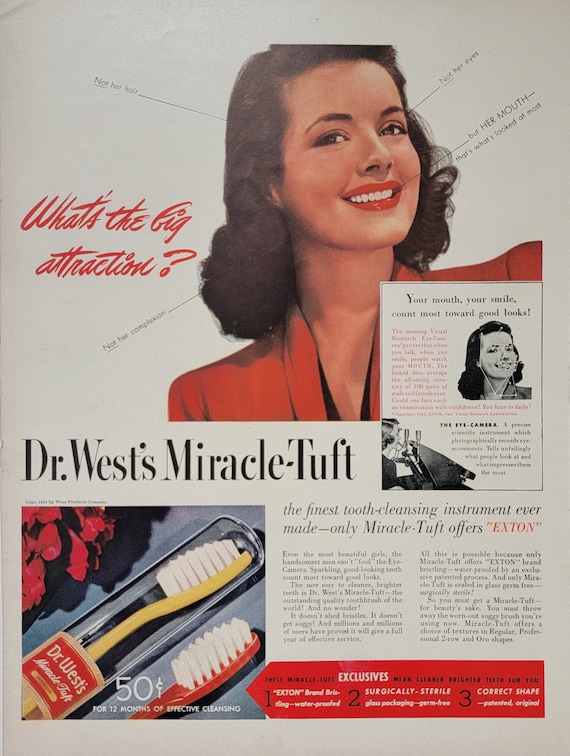This vintage advertisement for Dr. West's Miracle Tuft toothbrushes exudes nostalgic charm from the 1950s or 1940s. At the center of the ad is a radiant woman with dark, curly hair, styled in a period-appropriate manner, and a bright smile accentuated by red lipstick. She is elegantly dressed in a red blazer with a black-lined cleavage, embodying the era's fashion sense. To her left, a cursive script poses the intriguing question, "What's the big attraction?" Black lines radiate from her image to various facial features with annotations like "not her hair," "not her eyes," and "not her complexion," ultimately pointing out, "but her mouth. That's what's looked at most."

Beneath this focal image, the ad declares, "Dr. West's Miracle Tuft – the finest tooth cleansing instrument ever made," emphasizing that only Miracle Tuft offers the exclusive "Exton." A detailed illustration at the bottom left showcases two toothbrushes, one yellow encased in plastic and another red one, both priced at 50 cents for 12 months of effective cleaning. Adjacent to these toothbrushes, a red banner highlights three unique characteristics with an arrow pointing directly at the brush heads.

Additional text within the ad further elaborates on the benefits of using these innovative toothbrushes, reinforcing the overall message that a beautiful, healthy smile is the ultimate attraction.